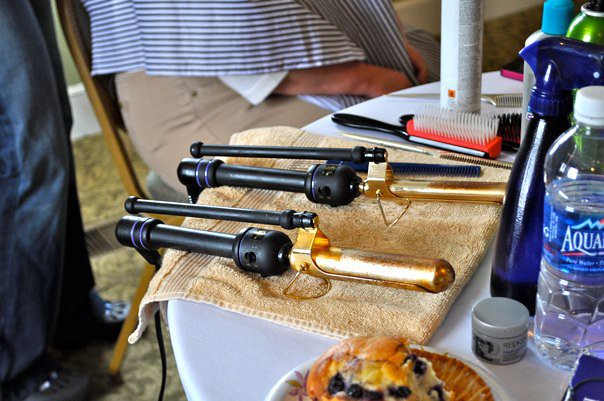The image captures a detailed scene of a hairstyling setup, likely in a home environment. At the center of the visual composition is a white table adorned with various objects. On the left side of the table lies a gold towel, upon which two curling irons rest. Both curling irons feature black handles with gold heating elements and clamps. Above them sits a hairbrush with a black handle, a pink inner base, and white bristles. Scattered along the right side of the table are several bottles, including an Aquafina water bottle, a small gray bottle, a taller blue bottle, and a green can partly peeking into the frame alongside a blue-topped container. In the lower foreground, there's an enticing blueberry muffin on a plate, partially eaten.

Beyond the table, a woman is seated in a gold chair, identifiable from her upper arms to her thighs. She wears a white shirt with sleeves that reach her forearms, over which a blue and white smock drapes down the front. Her hands rest in her lap over khaki pants. Behind her stands another figure, identifiable only by their blue jeans and black shoes. The overall scene suggests a personal, perhaps intimate hairstyling session taking place within a home setting.